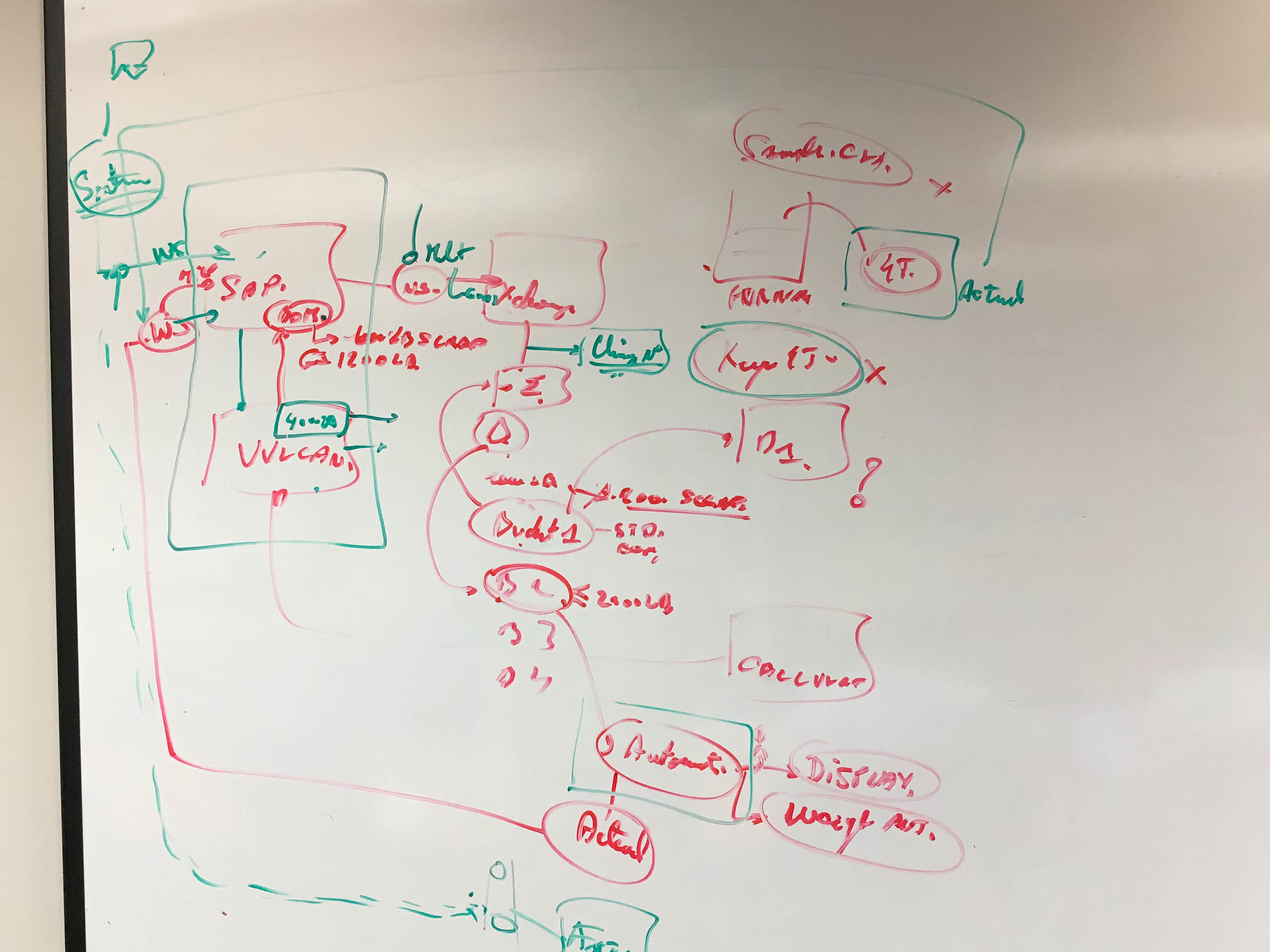The image depicts an old whiteboard densely covered with text and diagrams created using red and green markers. The primary focus appears to be a complex flowchart, though the exact subject remains unclear due to the illegibility of much of the text. The whiteboard surface shows signs of previous markings, indicating repeated use over time. In red marker, discernible words include "Vulcan," "Disney," "Simplicity" at the top portion, and "SOP" with an accompanying dot, likely an abbreviation. The green marker text also includes readable terms such as "Actual," and possibly "Net" and "China," though these are less certain. There's some visibility of the plain white wall surrounding the whiteboard, and a segment of its black framing is visible on one side of the board. The nature of the content hints at it being related to a scientific equation or a detailed flowchart, perhaps used for brainstorming or planning purposes.